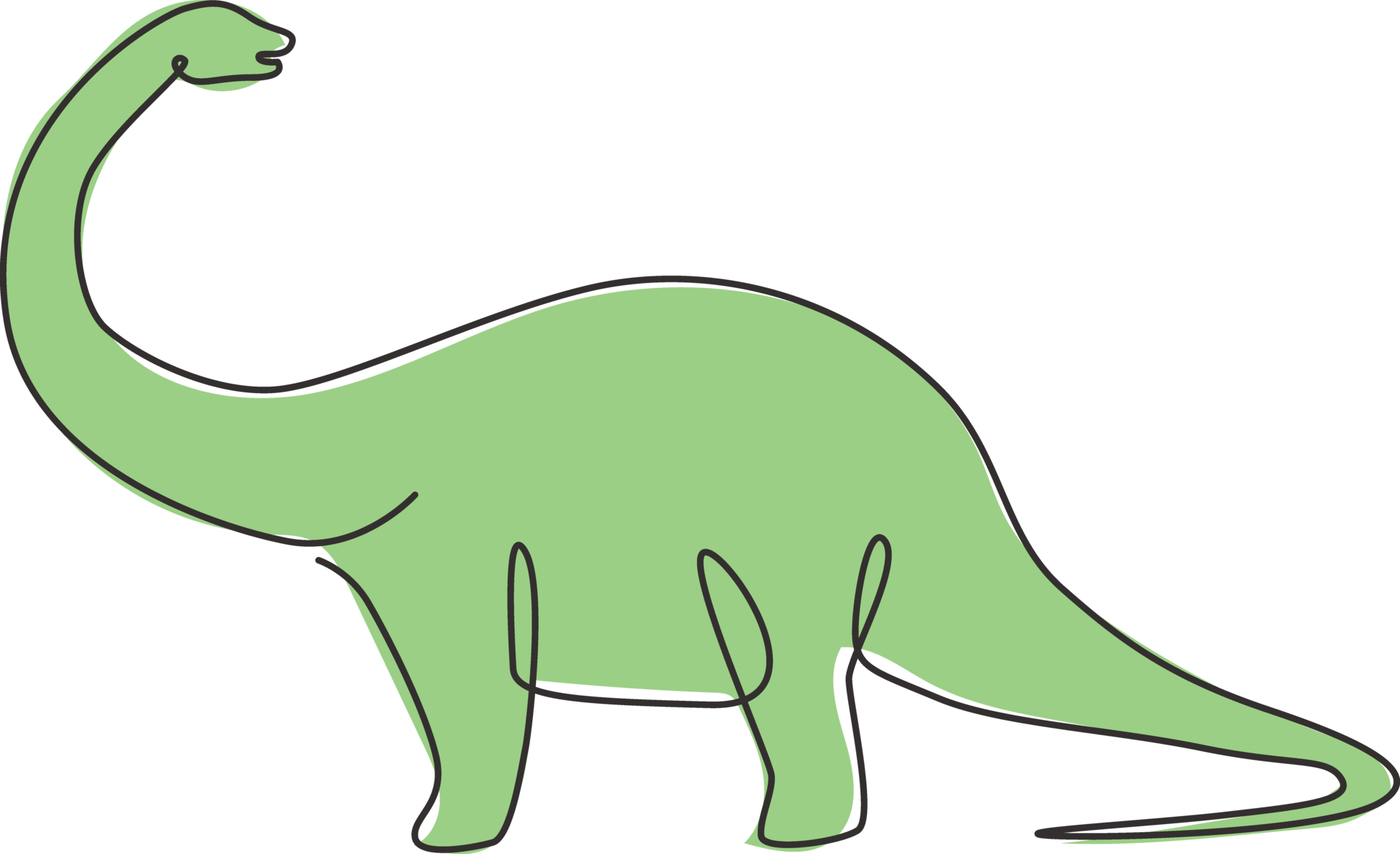This is an illustration of a long-necked dinosaur, likely a brontosaurus, rendered in a cartoonish, minimalistic style. The dinosaur is olive green with a single, continuous black outline that begins at the base of its neck and fluidly traces its form, looping around the head, down the neck, across the body, through the tail, and finishing at the legs. The drawing stands out against a white background and notably lacks facial features or intricate details. The green coloring does not completely fill the outline, leaving some white spaces, adding to its doodle-like, casual appearance. The dinosaur appears to be looking backwards, enhancing its impression of motion or curiosity. The creature is depicted with short, stubby legs and a long tail, giving it a simplified but charming look.